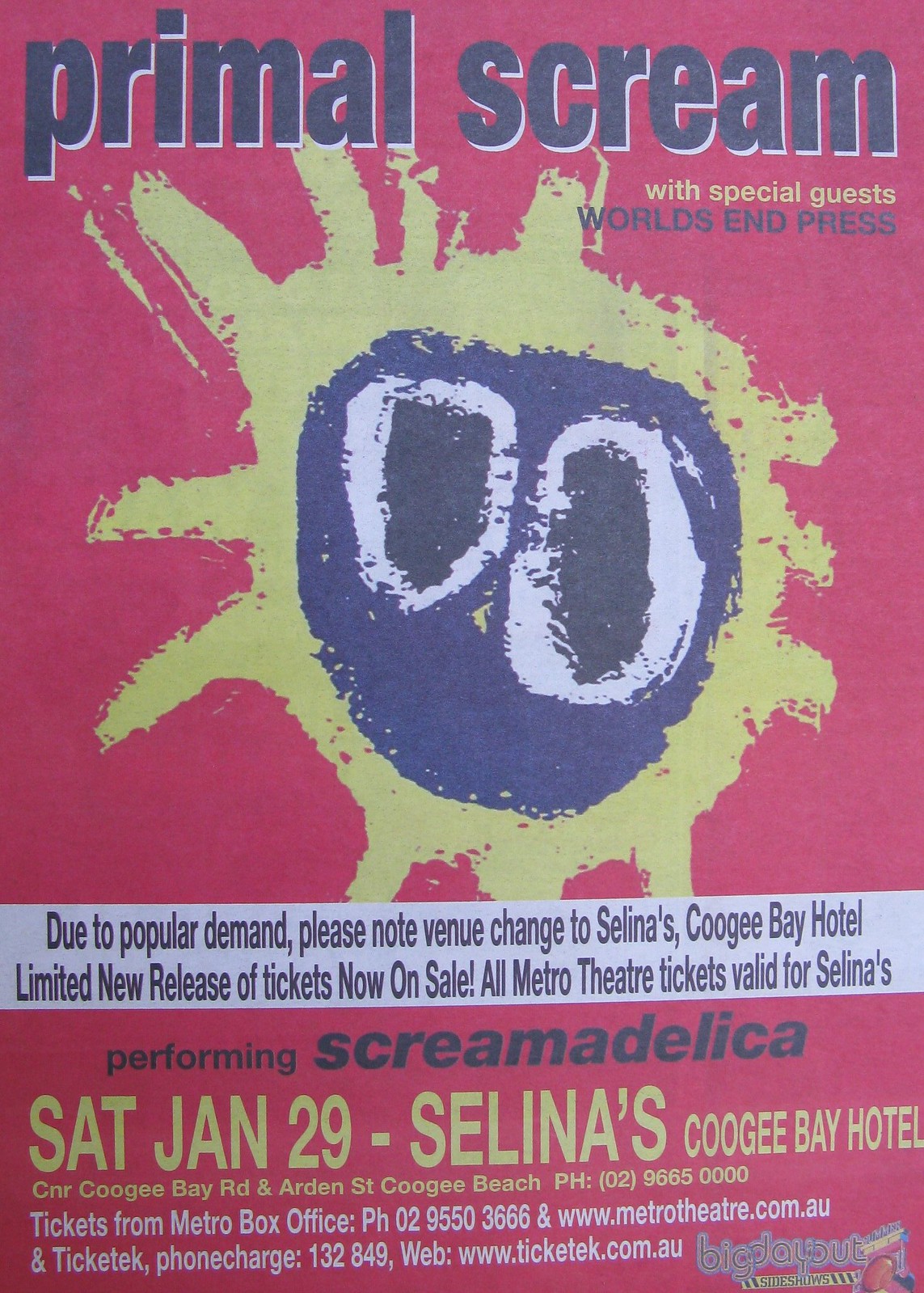The poster for the event has a vibrant red background with a striking, painted image in the center resembling a sun with a blue face featuring two large, sketchy eyes. This image gives the poster a distinctive, almost childlike appearance. At the top, in bold black text, it announces "Primal Scream with special guests, World's End Press." A white banner spans across the bottom of the sun image with crucial information: "Due to popular demand, please note venue change to Selena's Coogee Bay Hotel. Limited new release of tickets now on sale! All Metro Theater tickets valid for Selena's." Below this banner, the poster declares in black text, "Performing Screamadelica." Toward the bottom, it details the event date and location in yellow text: "Saturday, January 29th. Selena's Coogee Bay Hotel." Additional information about the venue's address, phone numbers, and ticketing details is also provided at the bottom of the poster.